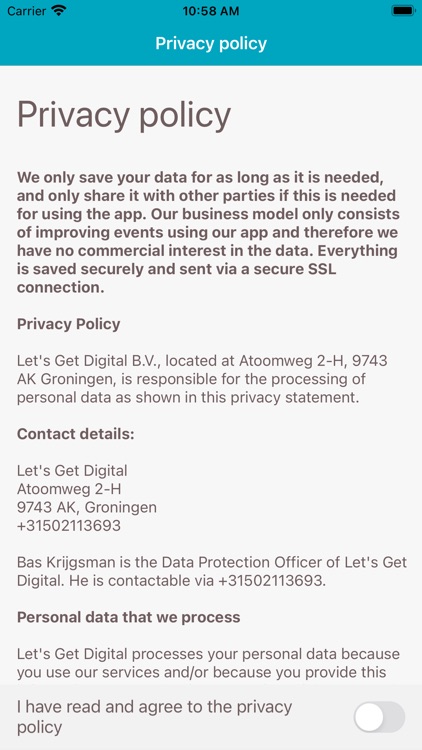The screenshot displays an app interface in portrait mode. The top part of the screen features a teal-colored header. On the upper left, the mobile carrier information is visible, while the top center shows the current time, 10:58 a.m. The upper right corner displays a full battery icon.

The first row below the header, still within the teal section, has the text "Privacy Policy" in white. The background below this header changes to a cream color. Centred in very large letters are the words "Privacy Policies." The following text explains: "We only save your data for as long as it's needed and only share it with other parties if this is needed for using the app. Our business model only consists of improving events using our app and therefore we have no commercial interest in the data. Everything is saved securely and sent via a secure SSL connection."

Further down, the sections are titled "Privacy Policies - Let's Get Digital VP," "Contact details - Let's Get Digital," and "Bass Krigsman is the Data Protection Officer." Another section, "Personal Data that We Process," follows.

At the very bottom, a slightly darker cream-colored row contains the statement "I have read and agreed to the privacy policy." To the right side of this statement, there is a toggle switch currently positioned to the left (off). To agree with the privacy policy, the user would slide this switch to the right, causing it to turn blue.